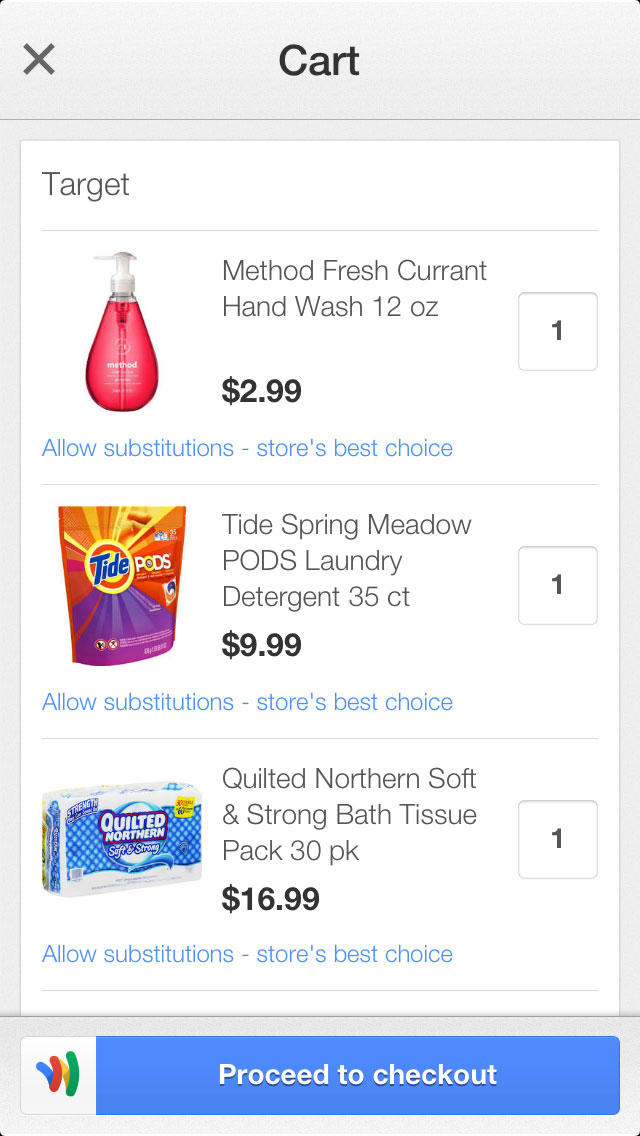Screenshot of a shopping cart from what appears to be a third-party grocery delivery app with a Target affiliation. The header of the app displays "Cart" in black text, and “Target” is noted at the top left, though the familiar Target color scheme is absent. Below the header, there is a list of items presumably being ordered for delivery. 

1. **Method Fresh Currant Hand Wash (12 oz)** - Priced at $2.99. An option for "Allow Substitutions" or selecting the store's best choice is visible, similar to Walmart's delivery service where substitutes can be chosen if the item is out of stock.

2. **Tide Spring Meadow Pods Laundry Detergent (35 count)** - The specific details including the number of pods and fragrance type are listed but the price is not mentioned.

3. **Quilted Northern Soft and Strong Bath Tissue (30 pack)** - Priced at $16.99. Again, the substitution options are available for this item.

The interface suggests a detailed order summary, with essential features designed to assure availability through substitutions, thus mimicking functionalities seen in other prominent grocery delivery services.